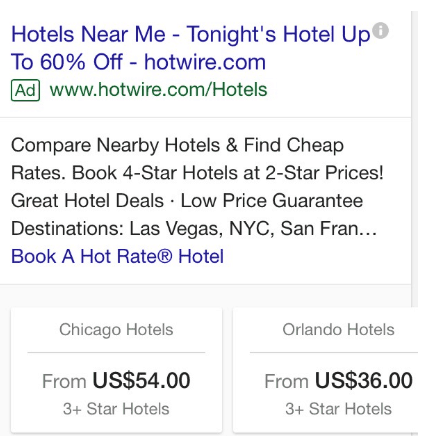This image captures a promotional advertisement for hotel bookings on a travel website. The background is predominantly white with a variety of text and elements organized across it. 

At the very top, there's a blue headline stating, “Hotels Near Me - Tonight’s Hotel Up to 60% Off - hotwire.com," hinting at significant discounts for last-minute hotel bookings. Positioned in the upper right corner is a gray information icon for additional details.

Just below the headline, there's a green box featuring the text “Ad” and a URL, “www.hotwire.com/hotels," indicating a sponsored link. A light gray bar separates this from the rest of the content.

Below the bar, black text encourages users to “Compare Nearby Hotels and Find Cheap Rates,” followed by the enticing offer, “Book 4-star Hotels at 2-star Prices. Great Hotel Deals.” It concludes with a point-form guarantee, “Low Price Guarantee,” and mentions some popular destinations like Las Vegas, New York City, and San Francisco.

Further down, there’s a blue call-to-action, “Book a Hot Rate® Hotel,” which is circled for emphasis. At the very bottom, the left side of the ad features listings for specific cities. For Chicago, it notes “Chicago Hotels” with a supporting gray bar, accompanied by pricing details in light gray and bold black text that reads “From $54,” and clarifies that these are “3+ star hotels.” 

Similarly, for Orlando, it showcases “Orlando Hotels” with similar design and pricing information, stating, “From $36,” and also specifying these as “3+ star hotels.”

The organized layout and strategic color use make it a detailed, user-friendly guide for finding discounted hotel deals.